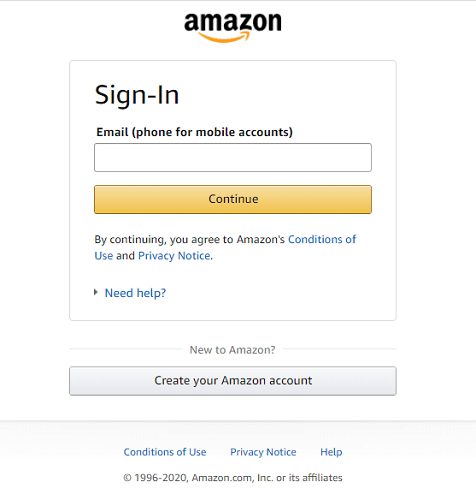Screenshot of Amazon Sign-In Page:

The image captures the Amazon sign-in screen, a familiar sight for many due to the widespread use of Amazon Prime and standard Amazon accounts. At the top of the screen, the iconic Amazon logo is prominently displayed with the word "Amazon". Below the logo, the heading "Sign-In" is bold and clear.

Central to the screen is an input box where users can enter their email address or phone number associated with a mobile account. Directly beneath this input field, a yellow "Continue" button invites users to proceed with the sign-in process. 

A disclaimer underneath the button informs users that by continuing, they agree to Amazon's Conditions of Use and Privacy Notice, both of which are hyperlinked in blue for easy access to the respective documents. 

At the bottom of the screen, a "Need Help?" button offers additional support options. Just below this, a message targets new users: "New to Amazon? Create your Amazon account." Accompanying this message is a grey button prompting the creation of a new account. 

The overall layout is clean, straightforward, and user-friendly, adhering to Amazon's consistently recognizable interface design.